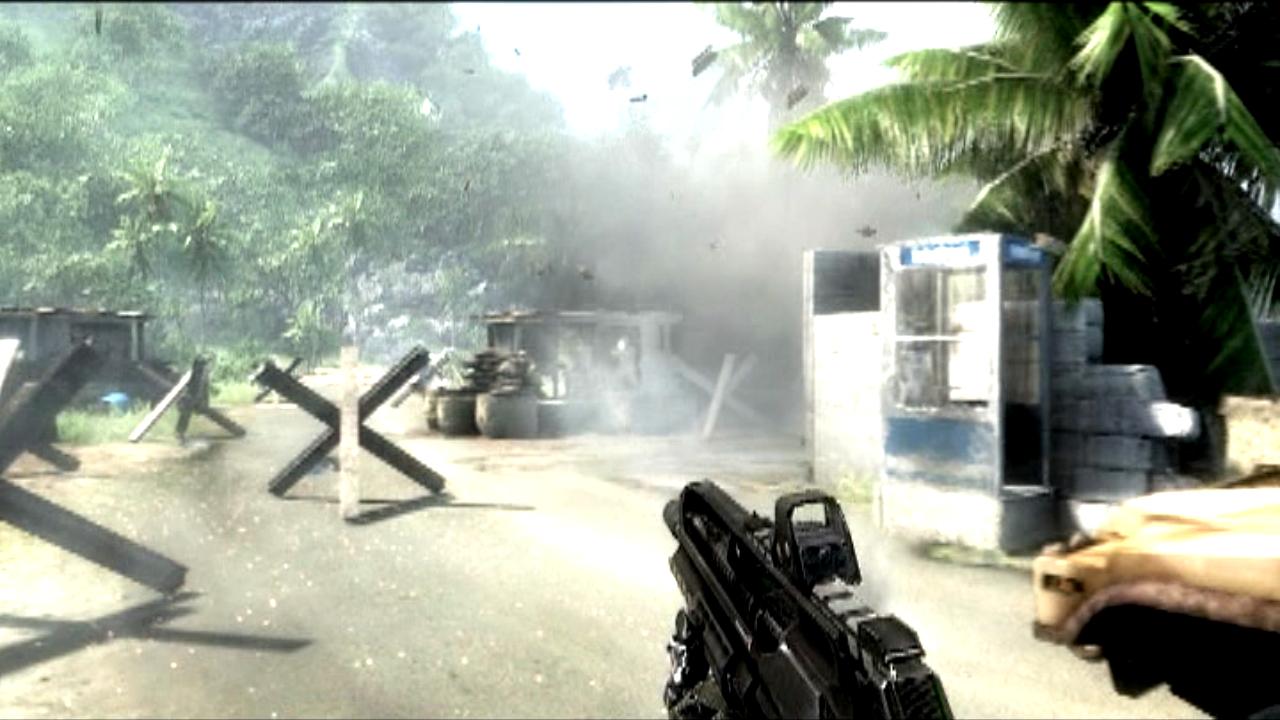The image, a still from a first-person shooter video game, presents a detailed and dynamic scene set in a tropical landscape. Captured from the protagonist's perspective, the foreground is dominated by an automatic rifle, its black barrel aimed slightly to the 11:30 direction. To the right, the bonnet of a Jeep or Humvee peeks into the frame, partially obscuring an old-school silver and blue phone booth topped by a towering palm tree. Multiple palm trees and other green foliage populate the background, contributing to the lush environment. The ground appears to be a mix of dirt and possibly short grass or asphalt, though it's not clearly defined. Central to the scene is a dirty grey blast cloud, likely from a recent explosion, with debris flying amidst the upheaval, indicating recent conflict. Just beyond the blast, a small hut sits near military-style barricades composed of large wooden beams forming X-shaped obstacles. To the left of the weapon's sightline, these barricades evoke the defensive structures seen on historic battlefields. A large hill looms in the top left corner, densely covered with palm trees and other vegetation, alongside a building nestled at the tree line. The overall image exudes a sense of tension and action, highlighting the juxtaposition of serene tropical beauty and the chaos of combat.